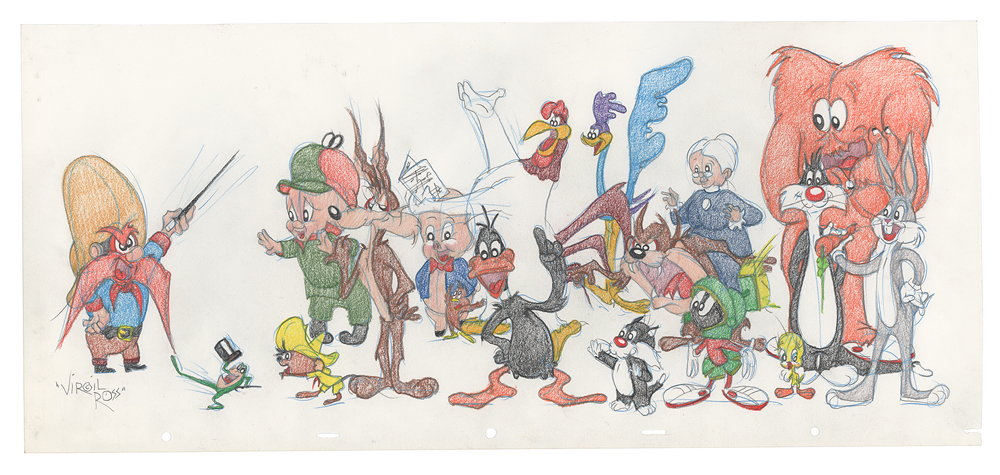The horizontal rectangular image, a detailed, colored drawing with a light gray background, showcases an ensemble of iconic Warner Brothers cartoon characters. At the left, Yosemite Sam, depicted as a conductor holding a thin stick in his left hand, directs the group. Below him, in small print, the name Virgil Ross signifies the artist. Just to Sam's right, a frog sporting a black top hat kicks his leg up in the air, followed by Speedy Gonzales in his yellow hat and outfit. Above Speedy, Elmer Fudd, clad in hunting attire, positions himself next to the slyly glancing Wile E. Coyote. Next in line is Porky Pig, donning a blue suit and bow tie.

Positioned a bit higher and to the right, Daffy Duck stands with one hand up, staring forwards. Behind him, Foghorn Leghorn appears engrossed in a book, his right hand raised as if singing or reading aloud. To Foghorn's right, the Roadrunner and the Tasmanian Devil occupy space near the image's center, with a small cat and a Martian below them. Tweety Bird is perched behind the Martian. Further back, Granny and a towering red blob-like creature, the Big Pink Monster, are visible. Sylvester the Cat stands in front of the monster, facing slightly left.

The right side of the image features Bugs Bunny, who is facing left, holding a carrot with a relaxed demeanor. This meticulously crafted drawing, likely executed with colored pencils, captures the essence of each beloved character, brought together in a lively scene, possibly a coordinated act or performance under Yosemite Sam's direction.